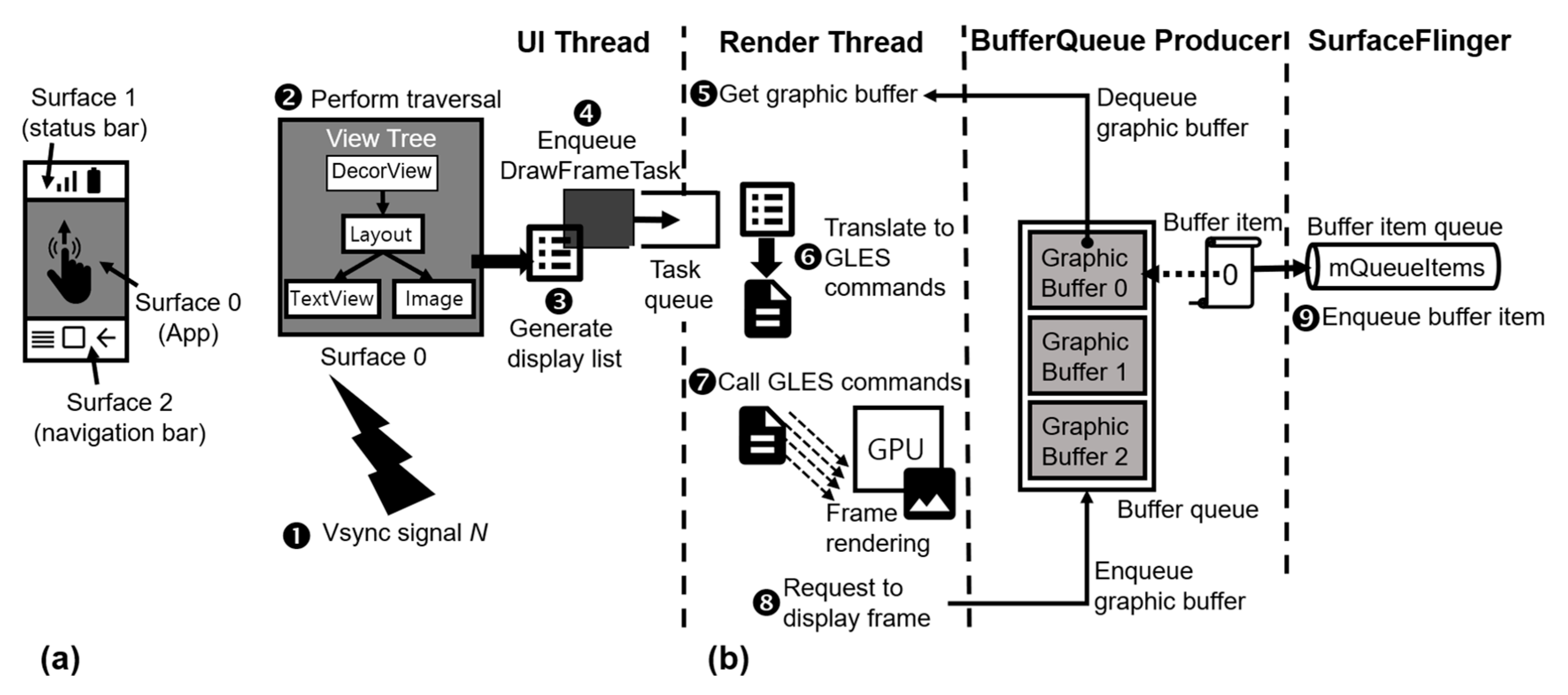The image is a detailed, black-and-white flowchart illustrating the intricate process of generating and displaying a graphical frame on a computer screen using a sequence of computational steps. Beginning from the left, the diagram starts with labels such as "Surface 1", "Status Bar", "Surface 2", and "Navigation Bar". It then complexly outlines processes involving the "UI Thread", "Render Thread", "Buffer Queue Producer", and "Surface Flinger", separated by dashed lines.

At the top, "Vsync Signal In" initializes the sequence, which leads to "Perform Traversal", encompassing subcomponents like "View Tree", "Decor View", "Layout", "Text View", and "Image". Following this, a sequence of tasks are highlighted: "Enqueue Draw Frame Task", "Generate Display List", progressing through a "Task Queue", and involving both the "UI Thread" and "Render Thread". 

The "Get Graphic Buffer" step retrieves buffers labeled "GraphicBuffer0", "GraphicBuffer1", and "GraphicBuffer2". These buffers are subsequently processed through "Buffer Queue" and "Producers", under the "BufferQueueProducer" section.

The flow then transitions through translating to and executing "GLES commands", with arrows indicating "Call GLES commands" leading to "Frame Rendering on the GPU". Once the frame rendering is complete, "Request to Display the Frame" ensues, resulting in the "Enqueue Graphic Buffer". These buffers cycle through labeled items such as "Buffer Queue", "GraphicBuffer", and "Buffer Item", finalized in the "SurfaceFlinger" with "BufferQueueItem" and "MQItems".

A rectangular graphic depicting a hand gesture and multiple steps involving arrows and connectivity, label the precise journey from initial signal to the final visualization, meticulously demarked.